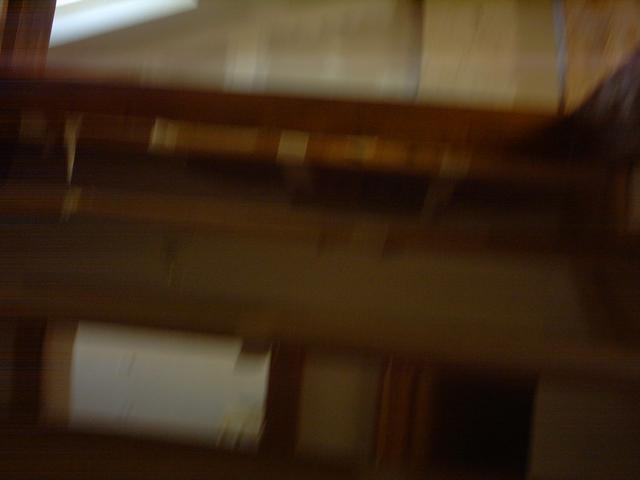This image appears to have been taken in a dimly lit environment, resulting in a highly blurred composition. The dominant colors are dark browns, light browns, and beiges, which contribute to the overall murky ambiance. It seems to depict an interior space, perhaps a room, where indistinct elements suggest the presence of walls and a ceiling. Particularly, a structure resembling the edge of a ceiling meets a wall, although the details are unclear due to the blurriness. In the bottom left corner, there is an object that might be paper, but it is too vague to accurately identify. The image’s lack of clarity leaves much to the viewer's imagination.